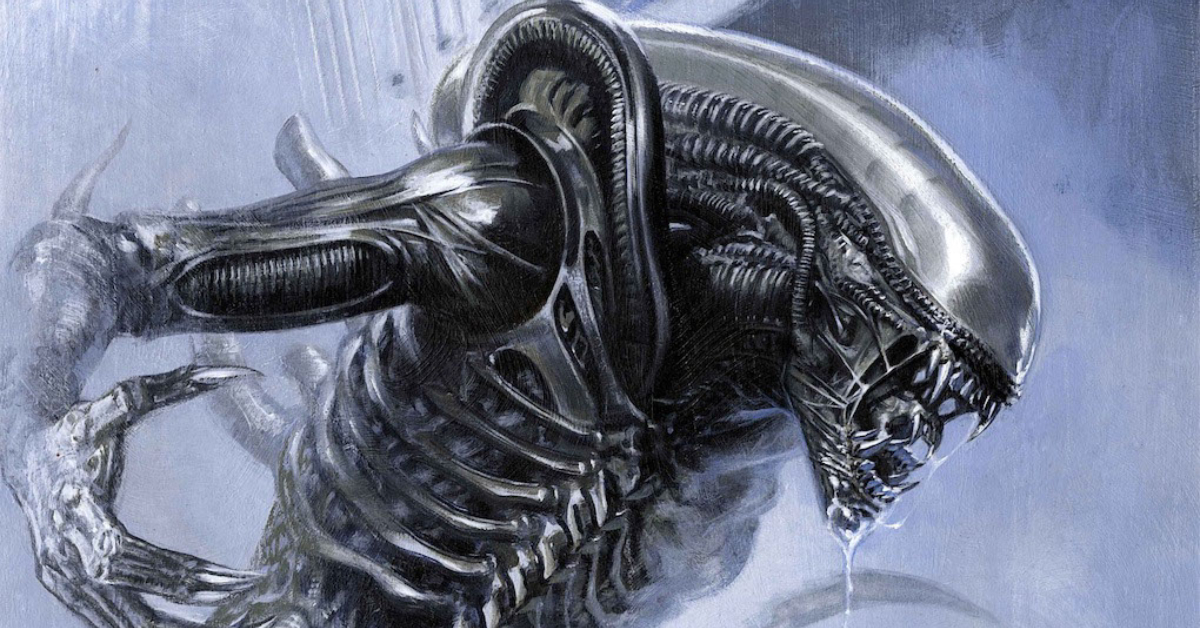This horizontally rectangular image is an artist's rendition of the iconic alien creature from the Aliens franchise, originally directed by Ridley Scott. The textured background features varying shades of gray, transitioning to a slightly darker tone in the upper right and a lighter patch on the left. The creature itself, depicted in a skeletal, metallic form, dominates the composition, its head and upper torso prominently visible. The creature's smooth, armored head, featuring corrugated tubes extending from its mouth towards its neck, gleams with a metallic sheen. The monstrous figure is leaning forward with menacing intent, its jaws open to reveal the smaller, inner mouth at the cusp of extending. Ribcage details and artery-like structures are clearly visible, enhancing its skeletal appearance. Its right claw, sharp and poised, is positioned towards the right side of the image, while the head angles menacingly towards the lower right corner. The overall gray palette emphasizes the creature's eerie, metallic exterior, making it the focal point of this chilling artwork.